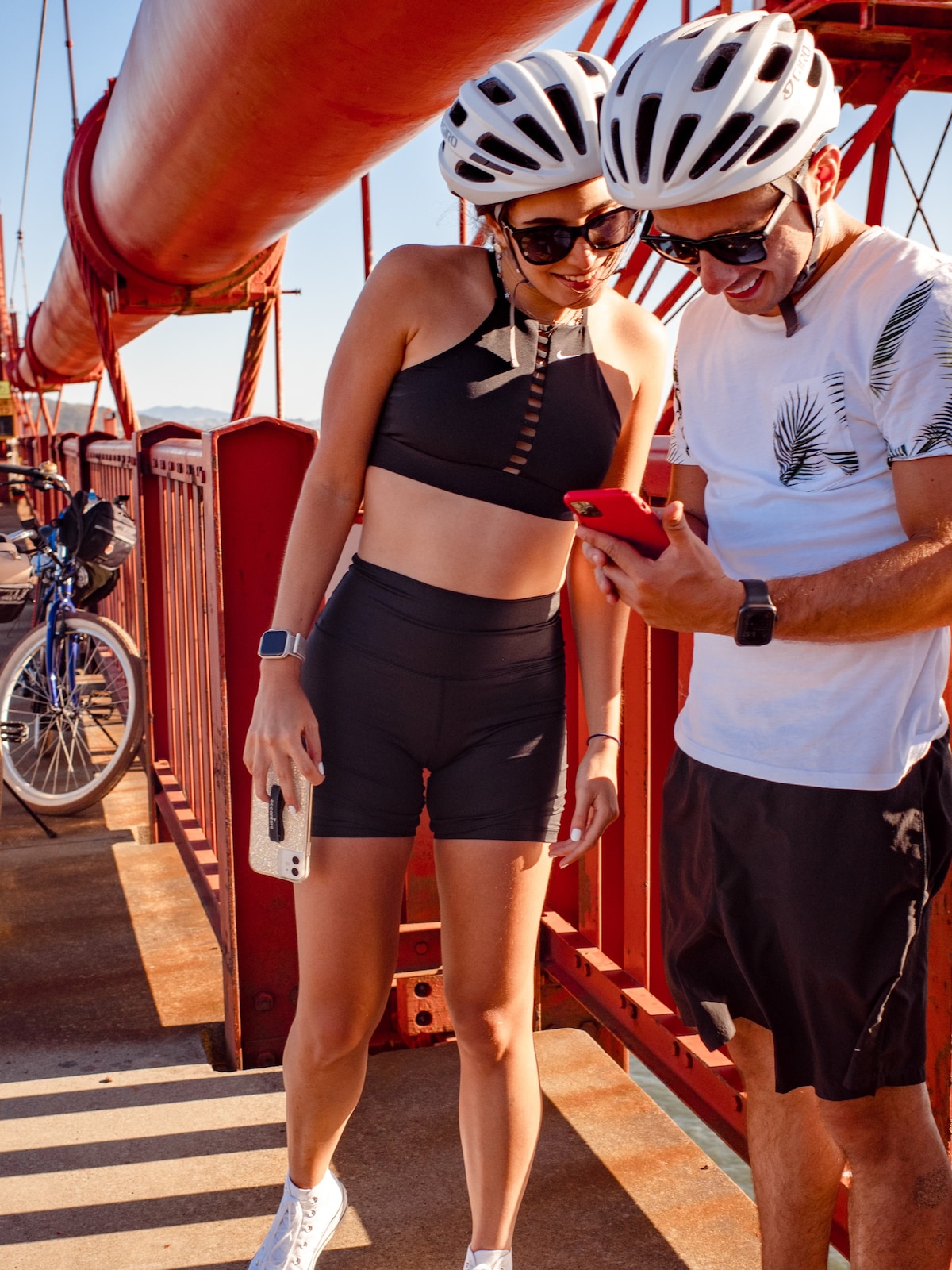On a bright and sunny day, a Caucasian couple is captured on a strikingly red suspension bridge with some rust on the railings. Both are wearing white bicycle helmets and black sunglasses. The woman, adorned with red lipstick, a black halter top, black shorts, and white tennis shoes, holds her phone casually at her side, her smartwatch on her right wrist. She's looking down at the man's red smartphone with interest, sharing a moment of enjoyment. The man, dressed in a white t-shirt with a design, black shorts, and sunglasses, is engrossed in his phone. The background reveals a blue bicycle and faint hills or mountains against a nearly clear light blue sky. The bridge's massive red piping and supporting beams accentuate the vivid structure, making the scene vibrant and dynamic.